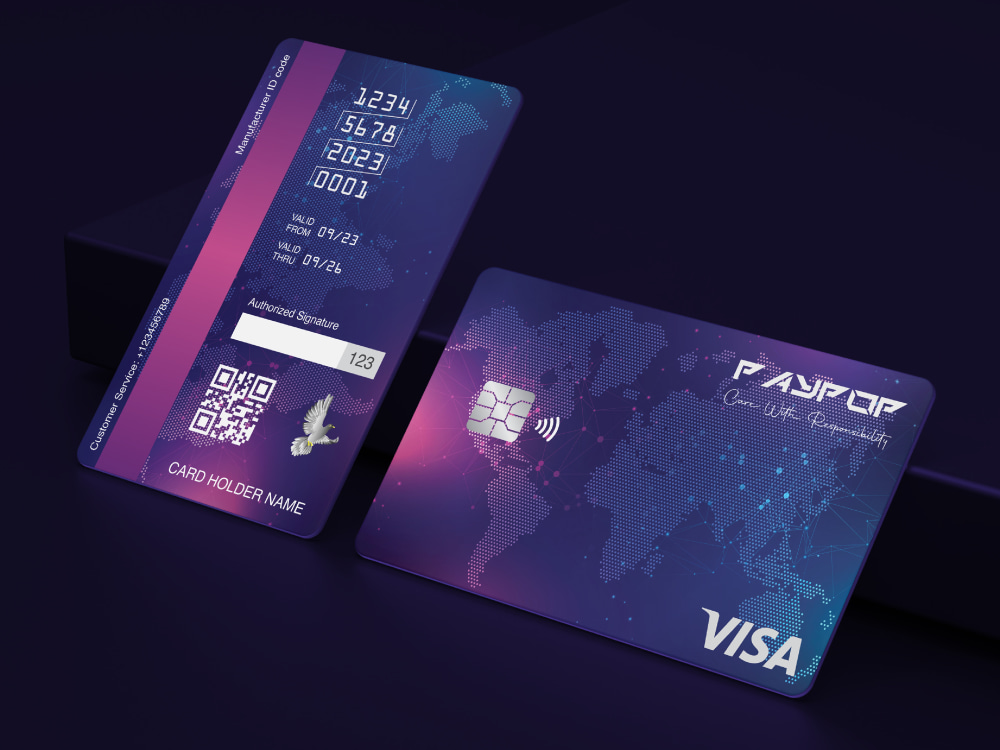The image displays a single Visa card photographed from both the front and back against a dark, purplish-black background. The card itself features a rich blue design with a dotted depiction of the world map. On the right side of the image, the front of the card is shown at a slight slant but remains horizontal. This side includes a silver chip on the left center, with a Wi-Fi symbol to its right, and the text "Pay Pop" and "I care with responsibility" near the top. The bottom right corner bears the Visa logo. The left side of the image presents the back of the card, vertically oriented. It displays a purple magnetic strip along the long edge and various details including: placeholders for the credit card number (1 2 3 4 5 6 7 8), a date code (2023 001), the valid from (09/23) and valid through (09/26) dates, an authorized signature strip with a white rectangular space for the signature, a three-digit security code, and a QR code at the bottom. Additionally, a bird logo, presumably an eagle, and the cardholder's name are also visible.